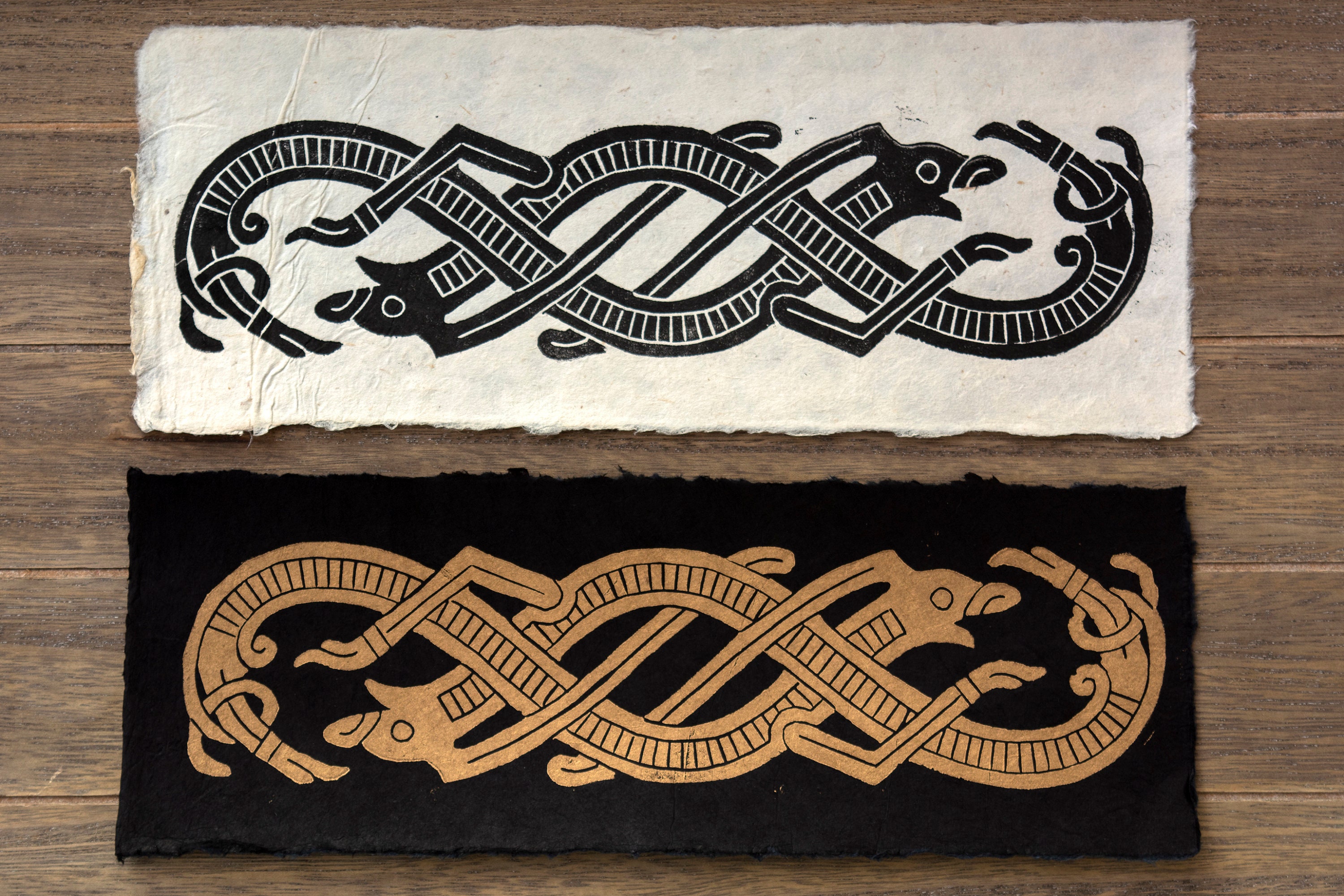This image captures two distinct yet similar pieces of art, displayed on a rustic wooden table. Each piece of art showcases a design featuring two intertwined creatures that resemble a mix of snakes and dragons, complete with intricate, detailed features such as beady eyes, open mouths, and arms emerging from their bodies. The top piece is printed on white pulpy paper with rough edges and depicts black creatures on a white background. The bottom piece, a black pulpy parchment, mirrors this design in a matte gold or light brown color against a black background, giving the impression of an inverted or complementary visual effect. The designs are richly detailed and evoke the aesthetic of Celtic art, with the intertwined forms resembling both serpents and dragons.